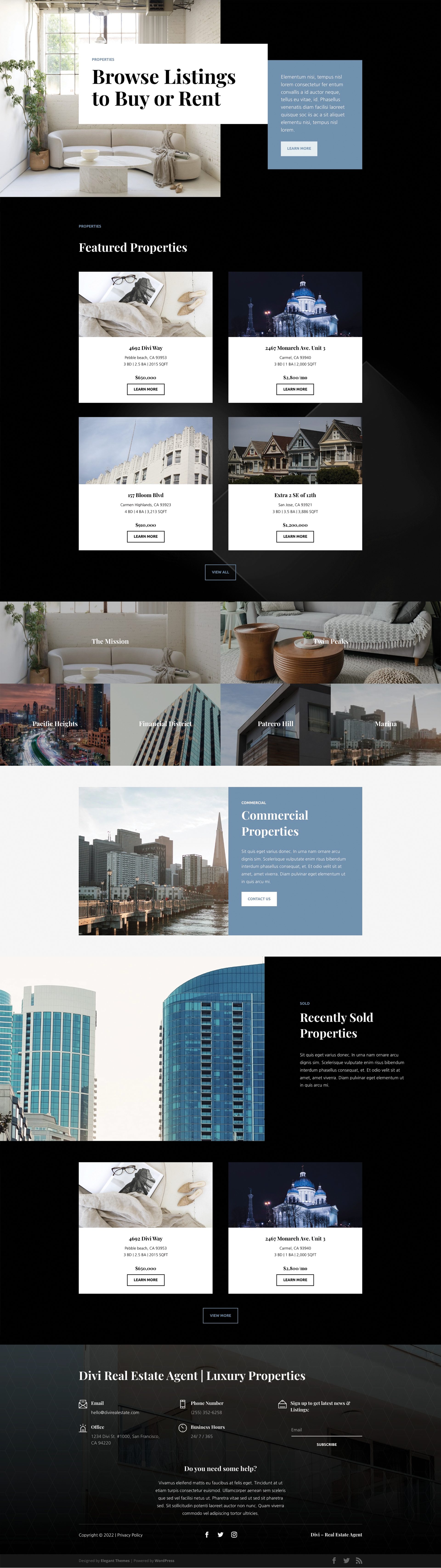This screenshot captures a comprehensive view of a modern, luxury real estate website, potentially named "Divi Real Estate Agent Luxury Properties." The website primarily caters to individuals seeking either rental or purchase options. The main navigation allows users to browse through available listings, segmented into properties for purchase or rent. Below this, the site showcases featured properties with four distinct high-quality images depicting lavish, upscale homes.

As you scroll further, the website reveals additional sections highlighting commercial properties alongside recently sold homes. Each listing is accompanied by white buttons for additional details, though the brief summaries beneath the headings are too small to discern. The overall aesthetic of the site is contemporary, with a sleek black background paired with white typography. High-resolution images dominate the visual layout, emphasizing the luxurious nature of the properties. The elongated nature of the screenshot suggests it might have been taken on a mobile device or from a zoomed-out perspective on a desktop, underscoring the site's high level of detail and user-friendly design.